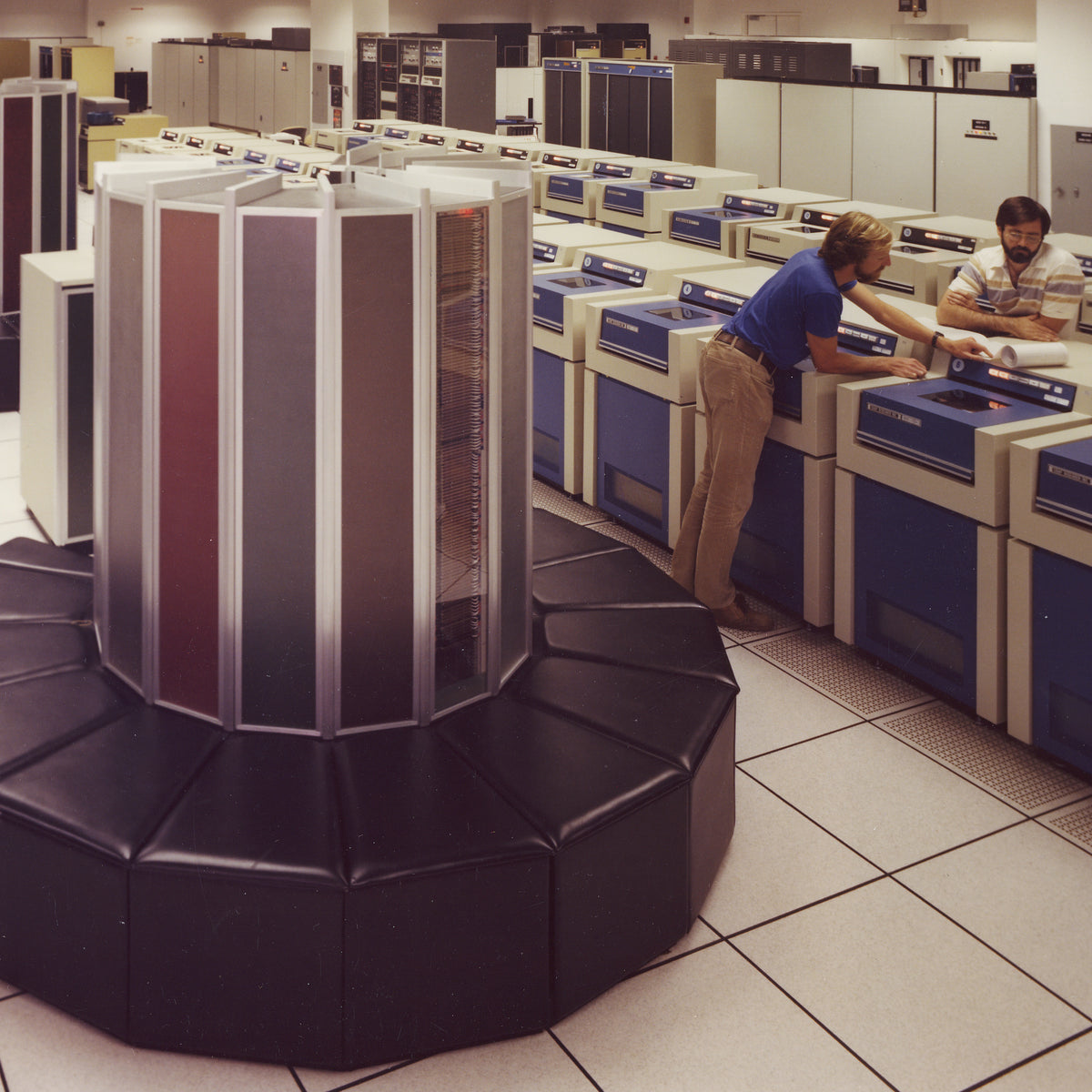This photograph, likely taken in the 1970s or 1980s based on the attire, captures the interior of a computer lab or scanning station. Dominating the scene are two men standing on either side of a large blue and white cubicle-shaped machine, resembling a washing machine but functioning as part of a computer data center. The machine features a glass-covered opening on top and a back panel with illuminated, albeit illegible, buttons.

The man on the left wears gray-brown corduroys, a brown belt, and a white polo shirt. He has shoulder-length blonde hair and a beard. Opposite him, another man in a striped polo shirt, with dark hair, a beard, and glasses, interacts with the machine, partially obscured by it.

The lab contains approximately 20 such machines arranged in two rows of 10. In the foreground, there's a unique circular seating area with black leather wedge-shaped seats surrounding a central cylindrical structure adorned with various rectangular vertical pieces. The background is filled with numerous cabinets and racks of indeterminate devices, adding to the technical ambiance of the setting. The tiled flooring, visible at the bottom of the image, reinforces the functional design of this vintage technological space.